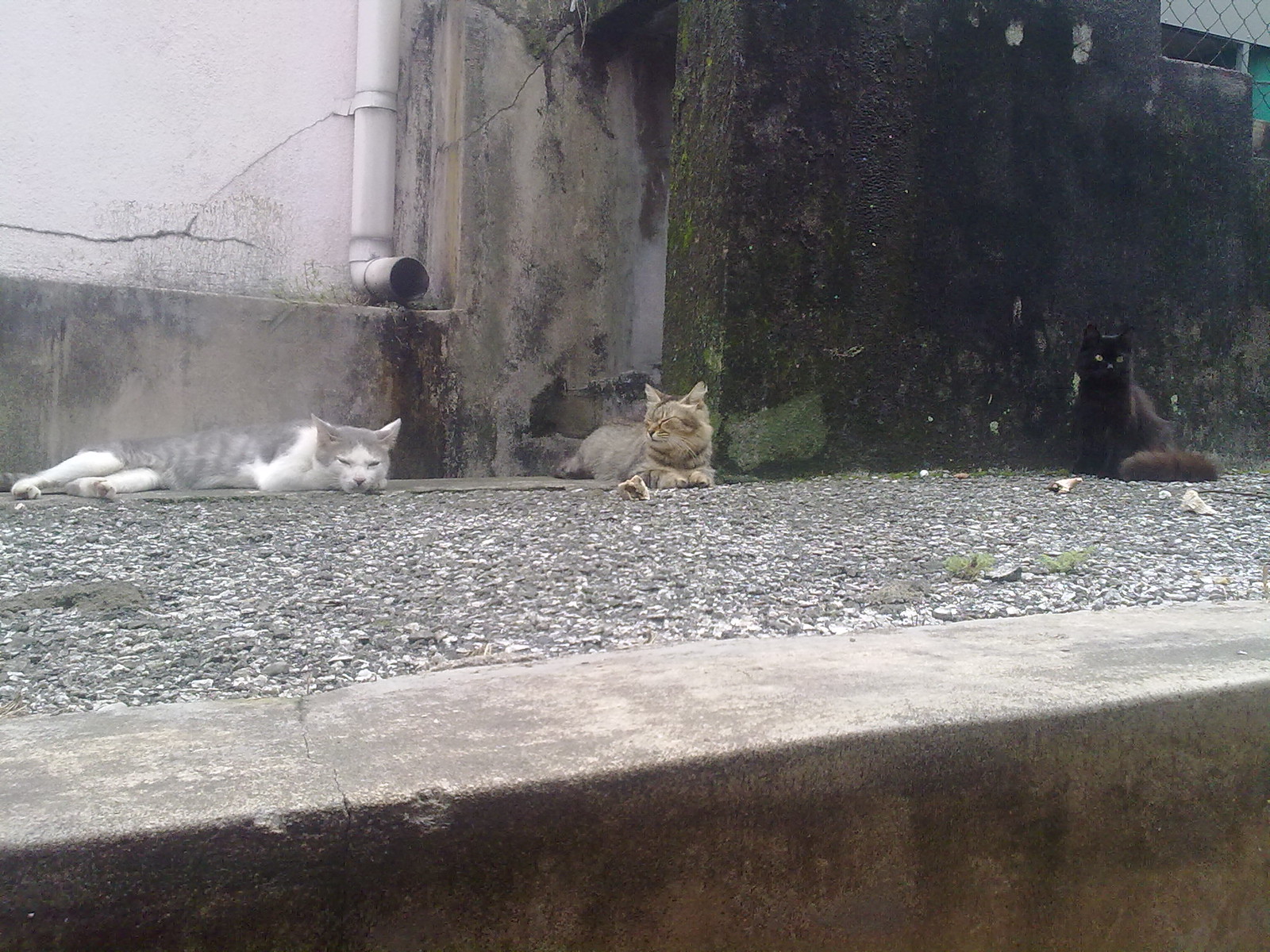In the image, we see an exterior scene next to an old building, likely situated in an alleyway or beside a street. The structure features a white wall marked with cracks and noticeable mold, indicative of persistent dampness. A prominent water spout runs down the wall, contributing to the moisture stains and mold growth. The wall finishes with a brown and black cement trim near the ground. The area below the wall consists of gravel with small stones scattered about, leading to a weathered walkway that edges into another part of the scene.

Three cats are present in this image. On the left, a gray and white cat lies on its side against the gravel. The central feline is a tan or light brown cat resting up against the building. To the right sits a black cat with a fluffy tail, blending into the darker segment of the wall. This cat appears alert, sitting upright in front of a section of the building that includes a barbed wire fence in the background. The setting exudes the rustic and weathered charm of an urban environment, with hints of greenery peeking through the gritty surroundings.